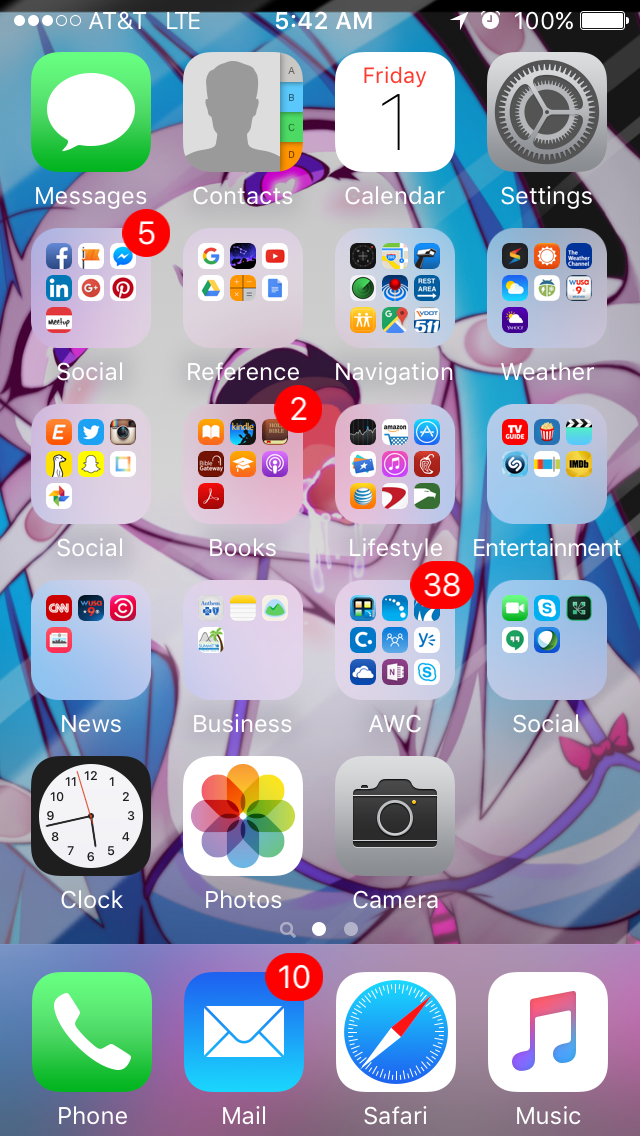This image appears to be a screenshot of an iPhone home screen taken at 5:42 AM. The status bar at the top indicates that the device is connected to AT&T’s LTE network, and the battery is fully charged at 100%. There are also indicators for location services and an active alarm.

**Status Bar:**
- Network: AT&T LTE
- Time: 5:42 AM
- Location services active
- Alarm set
- Battery: 100% and fully charged

**First Row of Apps:**
- Messages (Green icon with a speech bubble)
- Contacts (Gray icon resembling a contact book with a silhouette of a person)
- Calendar (White icon with the date "Friday 1")
- Settings (Gray gear icon)

**Organized Folders on Second Row:**
- Social (Contains apps like Facebook, LinkedIn, Pinterest, Facebook Messenger, with 5 notifications visible)
- Reference (Features Google Search icon among others)
- Navigation (Includes Google Maps and other navigation apps)
- Weather (Weather-related apps)

**Following Rows of Apps and Folders:**
- Books (Contains reading and ebook apps, 2 notifications visible)
- Lifestyle (Apps related to daily lifestyle)
- Entertainment (Apps for entertainment purposes)
- News (News-related apps)
- Business (Apps related to business activities)
- AWC (Unclear apps)
- Social (Another folder for social networking apps)
- Clock (Clock icon)
- Photos (App for viewing photos)
- Camera (App for taking photos)

**Bottom Row of Main Apps:**
- Phone (App for making calls)
- Mail (Email app, with 10 notifications visible)
- Safari (Web browser)
- Music (App for music playback)

**Background:**
- The wallpaper appears to depict an image in the hentai style of art.

Overall, the home screen seems well-organized with apps and folders sorted into relevant categories. The presence of multiple notifications indicates active usage of social media and email applications.